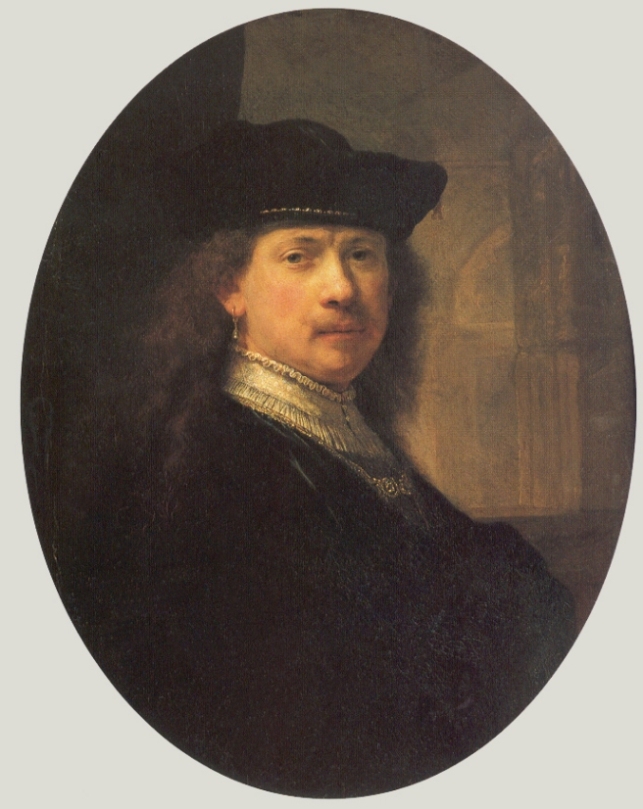This detailed self-portrait, likely of Rembrandt, features a mature and serious-looking subject, possibly a man, though certain features suggest a woman could also be portrayed. The figure gazes directly at the viewer, with a three-quarter turn of the body. The background is composed of a light gray square with an oval-shaped cutout framing the portrait, the backdrop of which includes different shades of brown, creating a subdued and indistinct scene behind the subject.

The person depicted has long, curly brown hair cascading down, and they wear a distinctive black hat, reminiscent of a beaver pelt, adorned with gold trim. The attire consists of a black overcoat, a high white collar ruffled below the chin, and a beautifully beaded necklace that merges seamlessly with the collar, suggesting elegance and a touch of opulence. There seems to be a faint wisp of a mustache adding to the ambiguity of the subject's gender. Completing the detailed look, faint silver earrings contribute to the refined aesthetic. The play of light strategically highlights the face, accentuating the serious expression and intricate details of the painting.